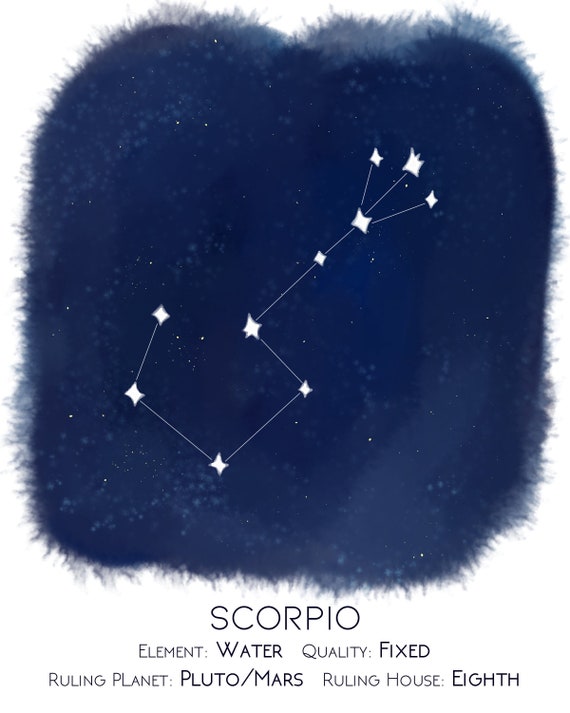This image features a detailed artistic rendition of the Scorpio constellation on a deep blue, pillow-like, furry object set against a plain white background. The constellation is illustrated with white diamonds connected by thin white lines, forming a scorpion-like pattern that culminates in a tail splitting into three segments. Below the blue object, the word "Scorpio" is prominently displayed in black text. Further down, additional textual elements in varying fonts and sizes provide astrological information about Scorpio, stating: "Element: Water", "Quality: Fixed", "Ruling Planet: Pluto/Mars", and "Ruling House: 8". The overall size of the image is estimated to be around five inches wide and four inches high. The blue pillow-like object adds a unique, soft, and tactile presentation to the constellation artwork, blending a sense of space with an almost tangible display akin to resting on furry material.